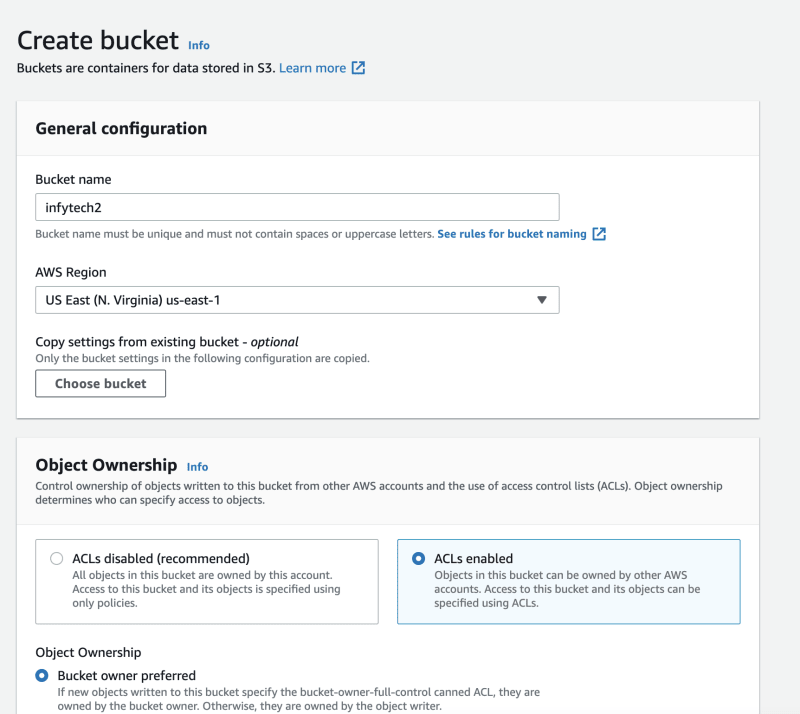The image is a detailed screenshot of the Amazon S3 bucket creation interface, set against a gray background. The primary heading in black text reads "Create Bucket," accompanied by an informational note. This note describes that "Buckets are containers for data stored in S3" and provides a link to "Learn more."

The interface is divided into several sections, beginning with "General Configuration." Here, the user is required to input a "Bucket name," which in this example is "INFYTECH2." Instructions specify that the bucket name must be unique, cannot contain spaces, or uppercase letters, with a link to "See rules for bucket naming." The "AWS Region" is currently set to "US East (N. Virginia) - us-east-1," selectable from a dropdown menu. There is also an optional section to "Copy settings from existing bucket," which clarifies that only specific configurations will be copied and prompts the user to choose an existing bucket.

The next section is "Object Ownership," which explains the control over objects written to this bucket from other AWS accounts and the usage of Access Control Lists (ACLs). Object ownership determines access permissions to objects.

Two options are provided in side-by-side boxes:

1. **ACLs Disabled (Recommended)**: All objects within the bucket are owned by the account creating the bucket, and access is controlled using policies only.
2. **ACLs Enabled**: Objects within the bucket can be owned by other AWS accounts, and access can be specified using ACLs.

At the bottom of the section, there is a note about "Object Ownership - Bucket owner preferred." It specifies that if new objects written to the bucket use the "bucket owner full control" canned ACL, they are owned by the bucket owner; otherwise, they are owned by the object writer.